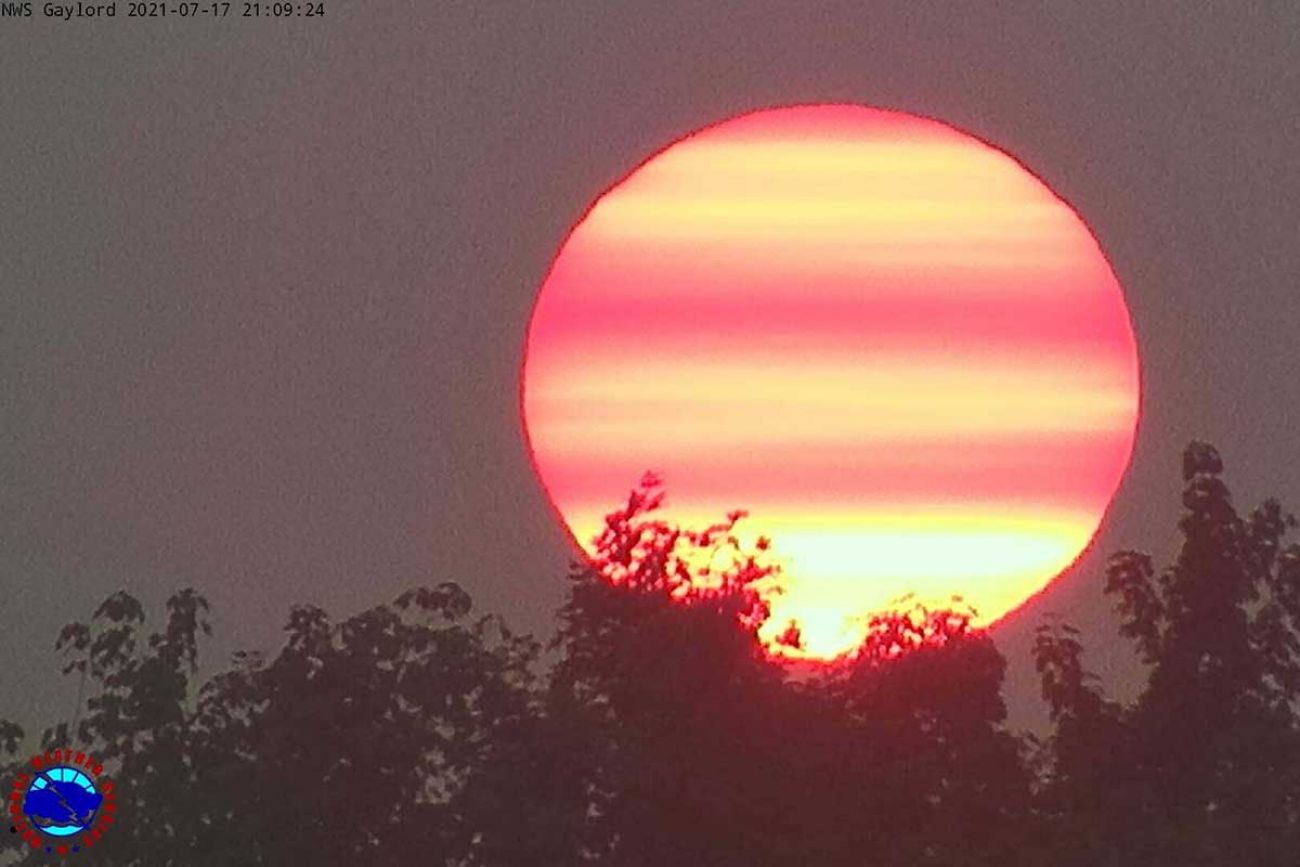This image captures a dramatic sun setting, with the sun's spherical outline distinctly visible. The background is a rich mixture of deep browns, grays, and reds, creating a surreal twilight atmosphere. The sun features multiple bands of color: red at the edges, transitioning through shades of light pinkish-red, darker pinkish-red, and several bands of light yellow, with a bright white area towards the center. Intriguingly, the sun is encircled by a dark red border, giving it an almost illustrated look.

In the foreground, there are silhouettes of tree branches and leaves stretching across the lower part of the image, adding depth and framing the celestial display. The bottom left corner contains a small, somewhat indistinct emblem with blue at its center and red text around it, indicating the image's possible source. Additionally, thin black text in the top left corner reads "NWS Gaylord 2021-07-17 2109-24," documenting the exact time and date, which enhances the photograph's mysterious yet precise nature.